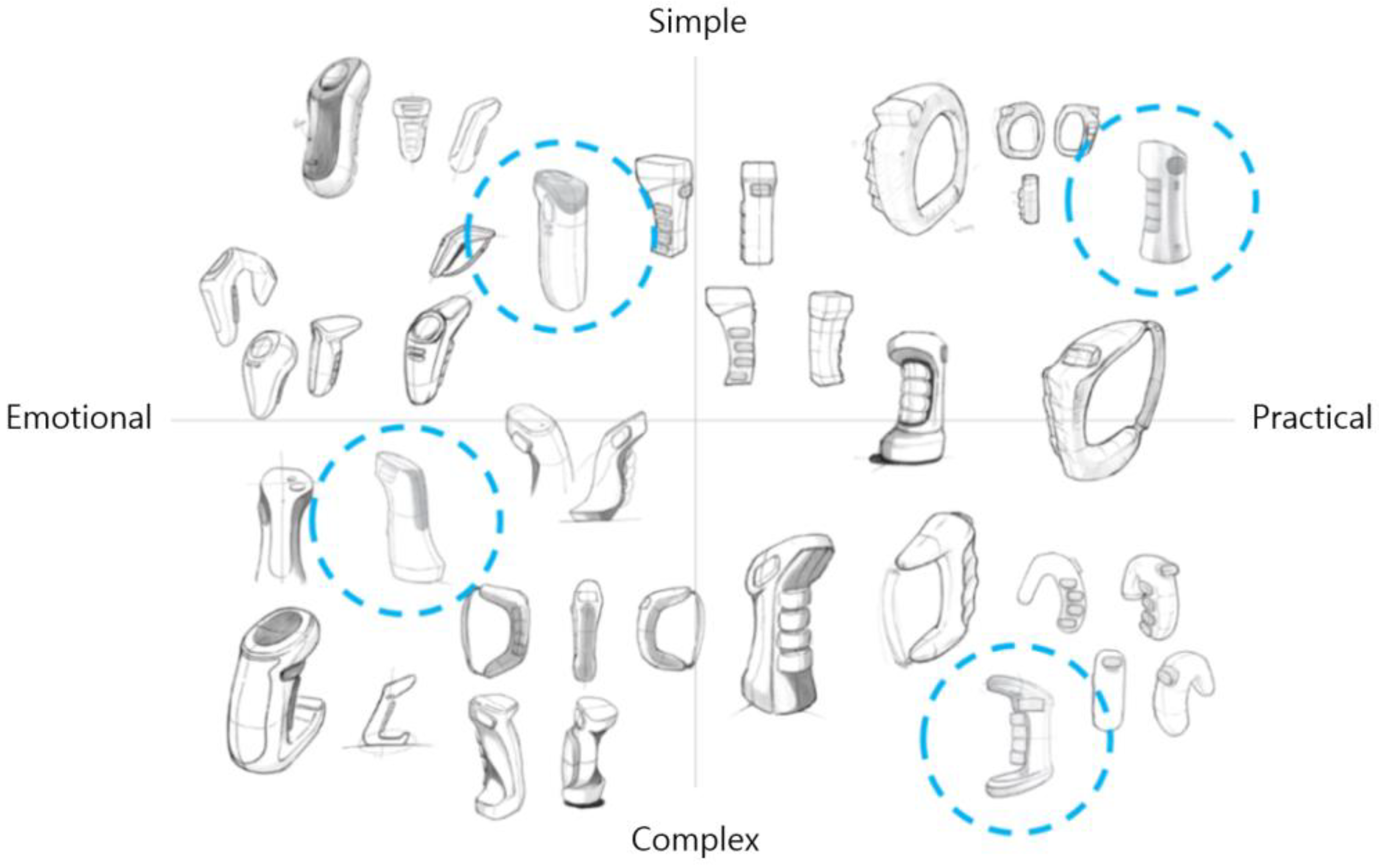The image is a detailed alignment chart featuring various illustrated joystick grips, arranged within a grid divided by light gray lines into four quadrants. Each quadrant is labeled with an axis name: "Simple" at the top, "Practical" on the right, "Complex" at the bottom, and "Emotional" on the left, oriented clockwise. All the depicted grips are pencil sketches and vary in design, with differences in texture, shape, and complexity. Some grips are smooth, while others are bumpy or elaborately curved; there are also simple stick-like designs. Each quadrant contains several joystick illustrations, with one joystick in each quadrant highlighted by a dotted blue circle. The image is set against a white background, enhancing the clarity of the detailed pencil illustrations.